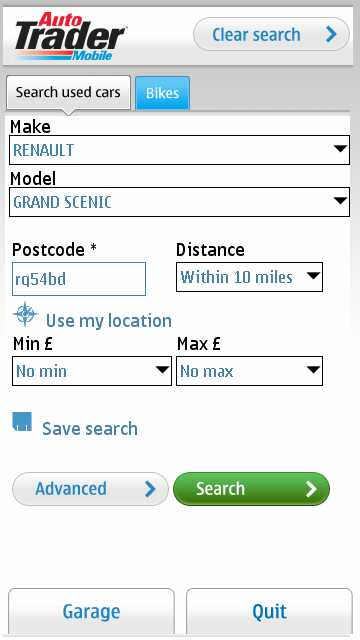In this image, which is a screenshot, the interface of a mobile app is displayed. 

### Upper Section:
- **Top Left Corner:** There is a gray banner featuring a smaller white banner. Within this smaller banner, "Auto Trader" is prominently written in red text, followed by "Mobile" in black.
- **Top Right Corner:** A search bar is located here with "Clear search" written in blue text next to it.

### Search Filters Section:
- **First Filter Row (Make and Model):**
    - *Make:* The label "Make" is displayed in black text. The adjacent drop-down box contains "Renault" in blue text.
    - *Model:* Below "Make," the label "Model" is shown in black text. The corresponding drop-down box contains "Grand Scenic" in blue text.
- **Second Filter Row (Postcode and Distance):**
    - *Postcode:* A box labeled "Postcode" displays "RQ54BD" as the entered text.
    - *Distance:* To the right, a drop-down box labeled "Distance" shows an option for "within 10 miles."
- **Additional Location Options:** Below these filters, there is an option labeled "Use My Location" featuring a compass icon.

### Price Range Section:
- **Price Filters:**
    - *Minimum Pound:* A drop-down box with an option for "No Min."
    - *Maximum Pound:* A drop-down box with an option for "No Max."

### Actions:
- An "Advanced option" button is provided for more detailed search parameters.
- A "Search" button is available to execute the search based on the selected filters.

This detailed description effectively captures the layout and elements present in the screenshot of the Auto Trader Mobile app's search page for used cars.